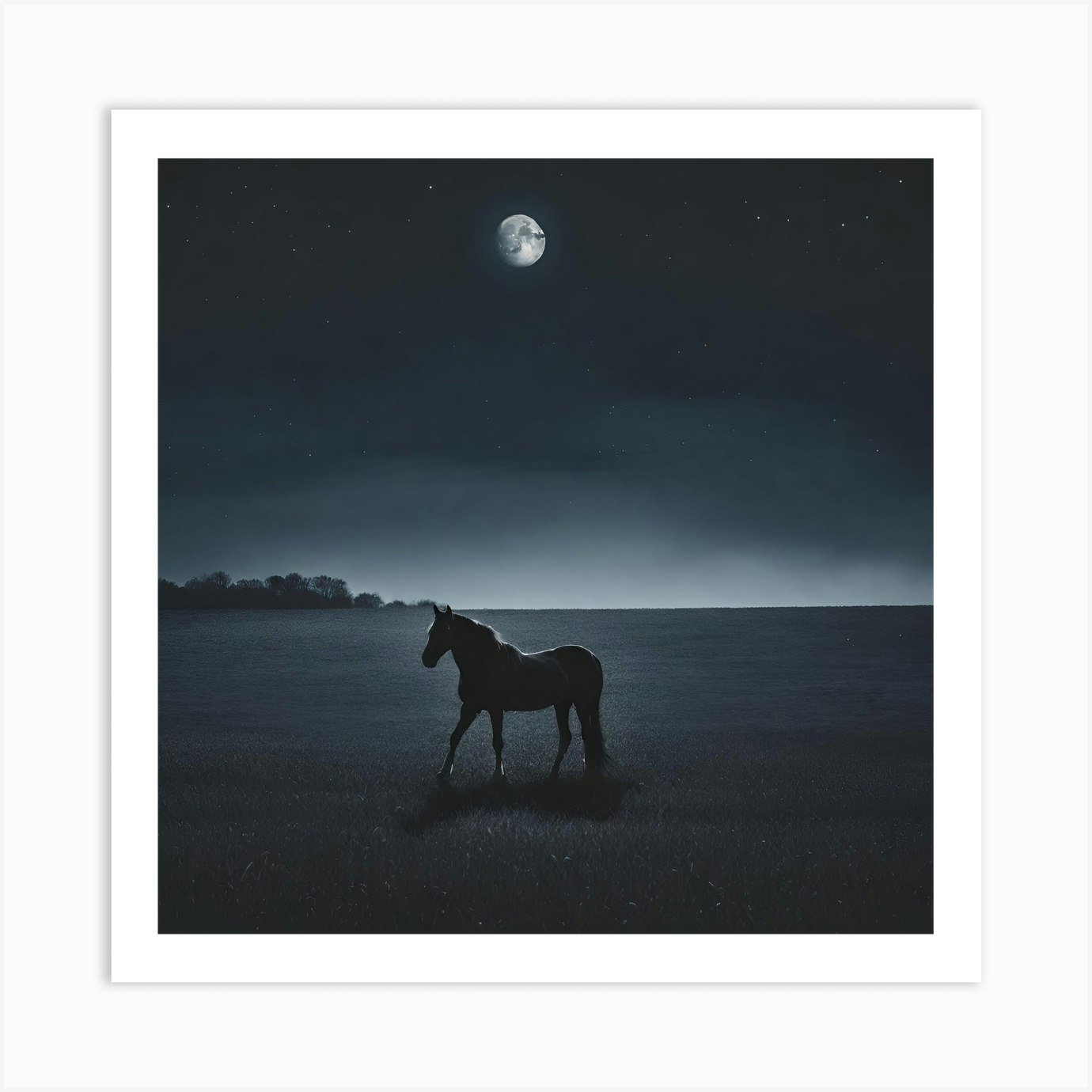The image depicts a night scene centered on a black horse with a white-topped mane, standing on a grassland. The scene is enveloped in darkness, making the horse’s facial features indistinguishable. The moon is prominently placed in the top-middle of the image, surrounded by a scattering of stars. The sky transitions from a deep black at the top to a lighter gray and near-white toward the ground level. On the left side of the horizon, low mountains are dotted with trees. The entire scene is contained within a square format, framed by a white border, giving it an appearance that oscillates between a digital image and a traditional photograph.